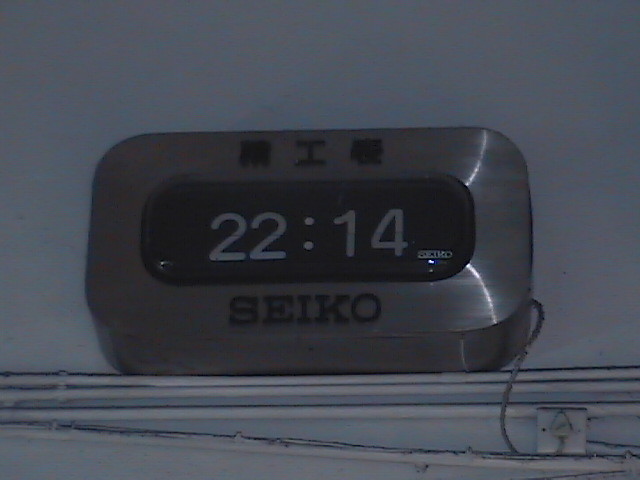In the image, we see a digital alarm clock. The clock is predominantly gray in color and features the brand name "Seiko" written in black lettering on the front, set against a black background. The digital display shows the time "22:14." The clock is plugged into a wall outlet using a black cord. Notably, there are three control buttons on the front of the clock, which are also gray. The image, although somewhat dark and unclear, allows the viewer to discern the brand and the time displayed. This device appears to be an alarm clock, possibly with radio functionality, and is likely placed in someone's home for timekeeping purposes.